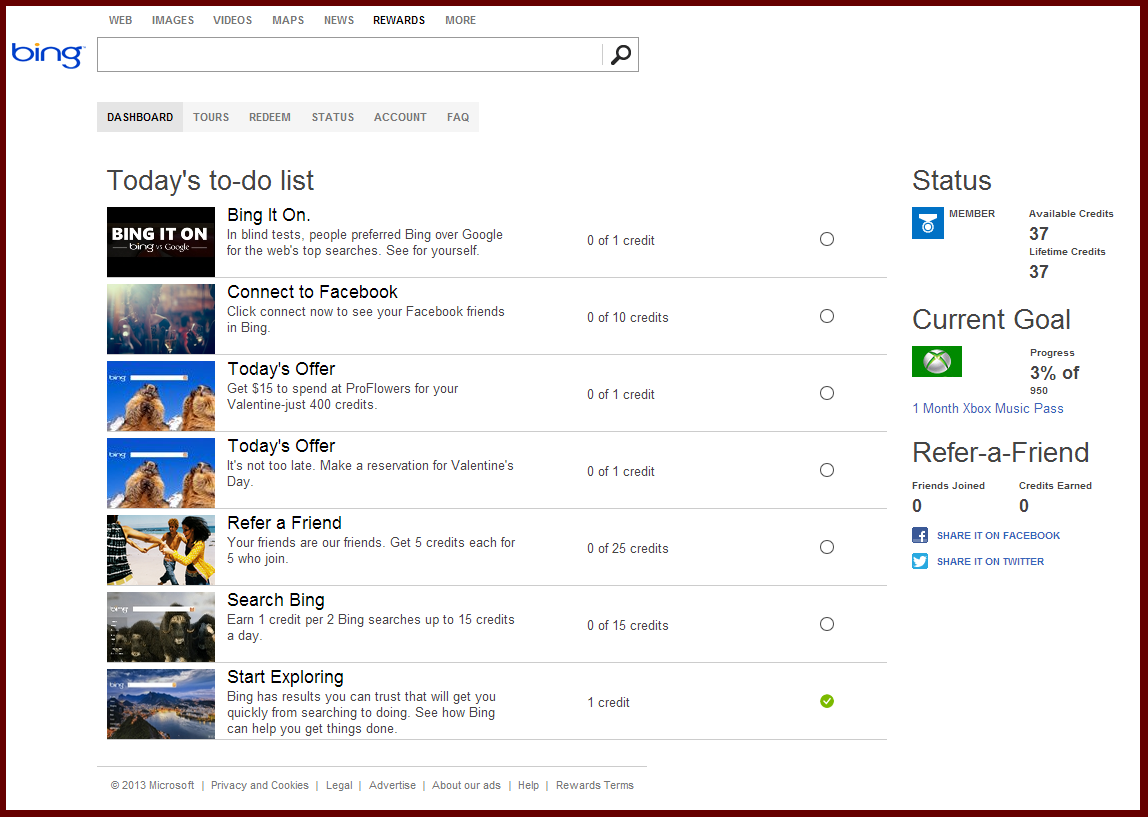The image showcases a large square with a thick mauve-colored border, featuring a white interior that appears to be the blank screen of a computer. In the upper left corner, the word "Bing" is displayed in blue text. Positioned above this are navigational options highlighted in black text, including "Web," "Images," "Videos," "Maps," "News," "Rewards," and "More."

Centered below these options is a search bar accompanied by a magnifying glass icon. Directly beneath the search bar, the text "Dashboard" is prominently grayed out, bolded, and selected, alongside other options such as "Tours," "Redeem," "Status," "Account," and "FAQ."

Scrolling down, the interface presents a "Today's To-Do List" section that includes pictorial icons and brief descriptions. One task, "Bing it on," invites users to compare Bing against Google in blind tests for the web’s top searches, offering zero credits for participation.

Additional tasks are listed, such as "Connect to Facebook," "Today's Offer," "Refer a Friend," "Search Bing," and "Start Exploring." The selected task, highlighted for emphasis, offers one credit.

In the upper right-hand corner, status information is displayed, indicating the user's membership status, 37 available credits, and 37 lifetime credits. The current goal's progress is depicted, noting 3% of 950 credits achieved. Options for referring a friend and sharing the status on Facebook and Twitter are also provided.